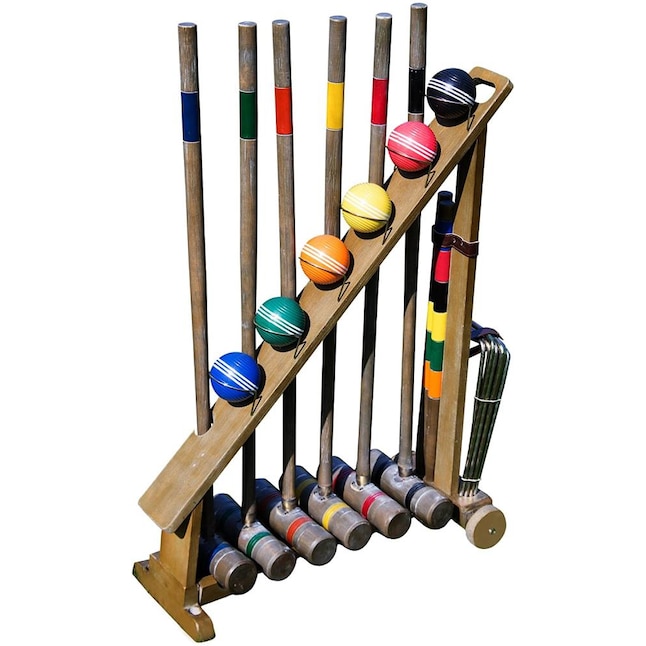This image showcases a detailed croquet set complete with a wooden storage holder designed for portability. The holder features wooden wheels at the back and a handle at the top for easy transportation. The front of the holder has a slanted board with compartments for six colored croquet balls—black, red, yellow, orange, green, and blue. The balls rest in metal brackets on this board. The set consists of six wooden mallets, each with distinct colored stripes around the handle and mallet head: three feature black accents, while the others display red, yellow, blue, orange, and green. In addition, there are metal stakes and hoops neatly arranged on the exterior of the holder, ready to be set up for a game. The overall design and organizational features of the holder ensure that everything needed for a game of croquet is readily accessible and easy to transport.